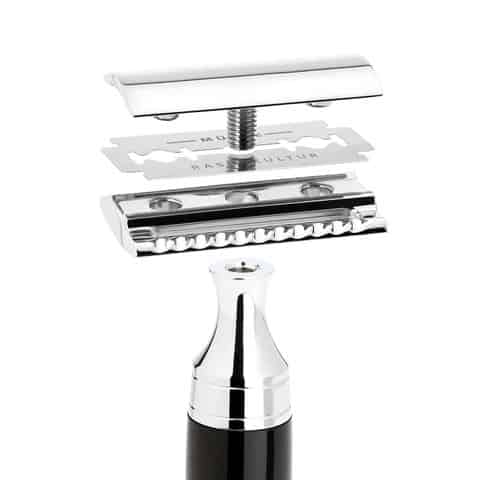This image is an extreme close-up, product shot often seen on Amazon, showcasing an old-fashioned safety razor against a white background. It highlights the construction and assembly of the razor, offering a detailed, exploded view of its various components. 

At the very bottom, a glimpse of the glossy black and silver handle is visible, while above it, three separated components of the razor blade section are prominently displayed. The handle leads up to a shiny chrome piece that bows inward, with a screw hole at the top. The first component above the handle is a metal bracket with three holes and beveled edges designed for smooth gliding against the skin. The middle part is the razor blade itself, featuring holes for alignment and a circular hole for the screw. The topmost piece is a rounded, chrome-finished cap with a screw attached, which ultimately goes through all the layers to secure the blade in place when assembled.

This detailed depiction, set against a white backdrop, serves to illustrate the internal structure and functionality of the safety razor, emphasizing how the parts fit together seamlessly.